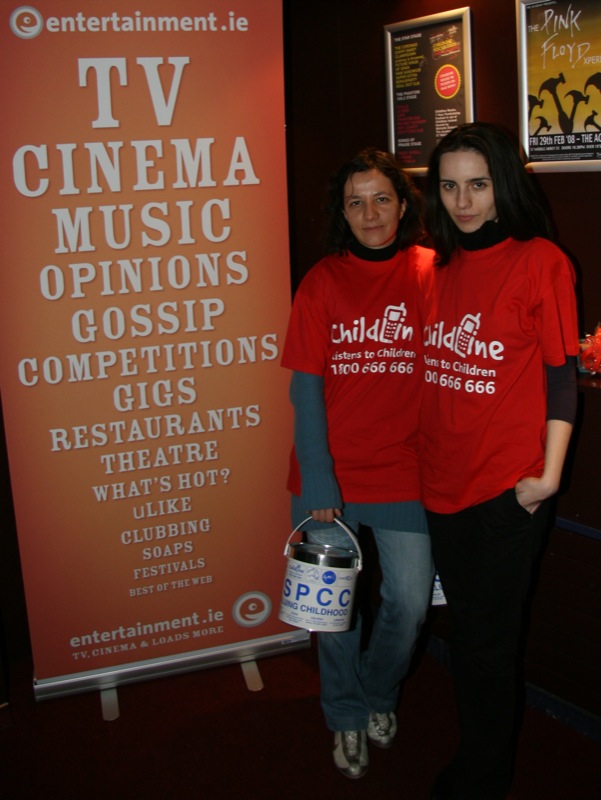The photograph captures a somber scene of two women standing slightly right of center, posing inside a dimly lit space against a backdrop of entertainment-themed posters framed in silver. Each woman is wearing a distinctive red t-shirt emblazoned with "Child Line" and the slogan "Sisters to Children," along with the phone number "1-800-666-666." 

The woman on the left, appearing slightly older, has short, reddish-brown hair and outfits a dark blue, long-sleeved sweater underneath her t-shirt. She is dressed in blue jeans and sneakers and holds a white metal donation bucket labeled "SPCC." 

Standing next to her, the younger woman on the right sports shoulder-length black hair and pairs her red t-shirt with a skin-tight top underneath and black pants, though her shoes are obscured. 

Beside the women, a brightly emblazoned orange banner promotes "entertainment.ie," listing various forms of entertainment such as TV, cinema, music, opinions, gossip, competitions, and more, in vivid detail. Despite the lively background, the women display a serious demeanor, adding a poignant note to the scene.